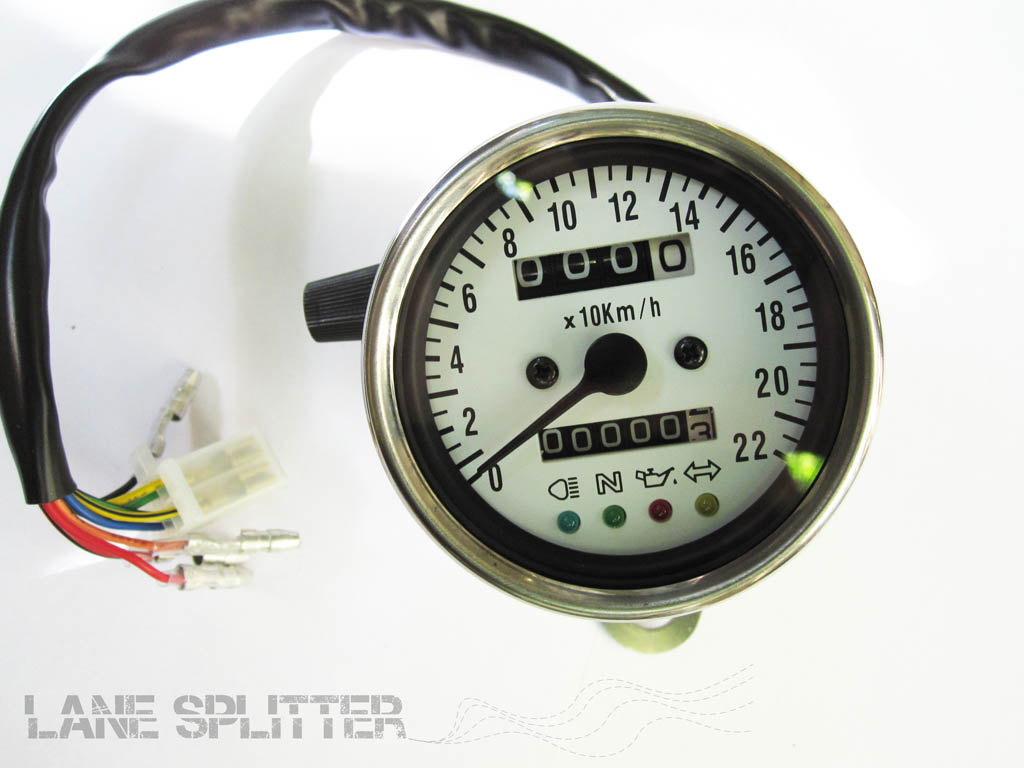The image depicts a vehicle dashboard device, specifically a combination instrument cluster that provides various pieces of information to the driver. At the top of the circular display, a speedometer starts from 0 at the center-left and increments up to 220, enclosing the top half of the display. This speedometer uses a series of numbers arranged in a semi-circular pattern along the edge of the circle. 

At the bottom-center of the circular display, there's an odometer that shows the total distance traveled by the vehicle using a series of rotating numbers housed in a rectangular window. Above the odometer, four indicator lights are positioned, each signifying different vehicle statuses. These include, from left to right, a warning light, an engine indicator, a fuel gauge icon, and a dual-ended arrow which most likely represents the turn signal indicators. Below these lights, the illuminated indicators show their current status, providing visual cues for the driver.

Overall, the intricate design of this instrument cluster ensures that a variety of essential driving metrics and warnings are conveniently displayed in a coherent and accessible manner.